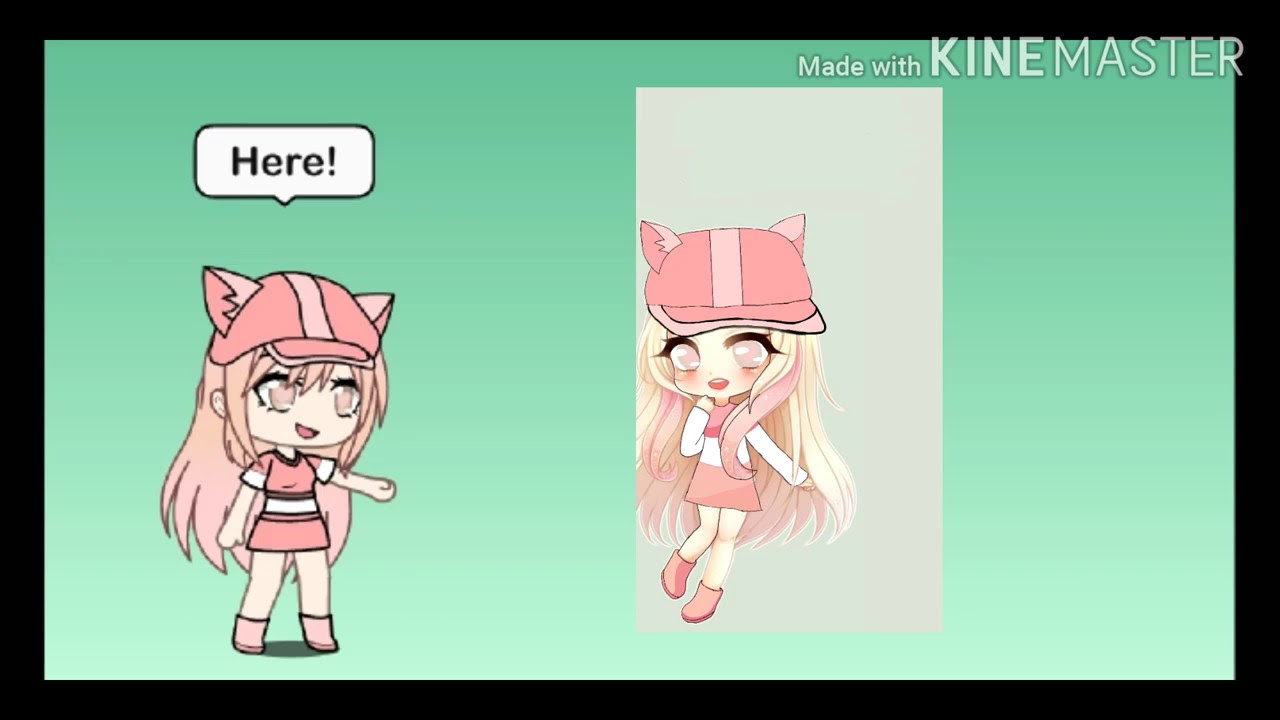The image is a rectangular graphic with a black frame, featuring two cartoon anime avatars of a female character. The top right corner of the image displays the text, "Made with KineMaster," with "Kine" in bold, against a minty green gradient background. On the left side of the image, the character appears with long pink hair, pink eyes, and pink ears on a pink ball cap. She wears a pink and white crop top, a pink skirt, pink boots, and has detailed eyeliner and blush. Her mouth, shaped like a wedge, is also pink. She has an outstretched arm and a speech bubble above her head that says, "Here!" with an exclamation point in black letters. On the right side, a mirrored, more detailed version of the same character appears against a beige gradient background, without any caption.